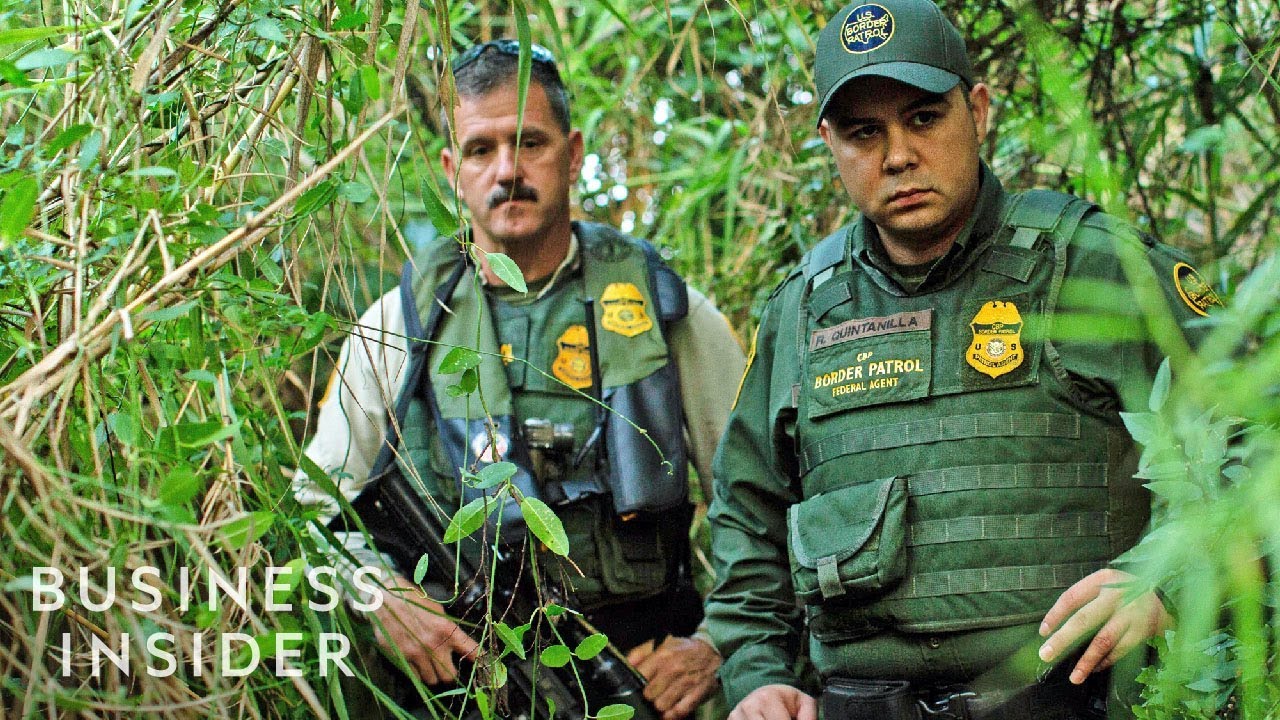The image is a horizontally aligned rectangular close-up photograph of two Border Patrol agents traversing a dense, semi-tropical forest area filled with various shades of green foliage, including twigs, leaves, dry branches, reeds, oval-shaped leaves, and palm fronds. The only visible sky is a small, bright patch in the center of the frame. In the lower left corner, the text "BUSINESS INSIDER" appears in all capital white letters, stacked vertically.

On the left side of the image stands a male agent who appears to be in his fifties. He has short, salt-and-pepper hair, a mustache, and is wearing sunglasses on his head. His uniform consists of a tan long-sleeved shirt under an olive-green with blue-trimmed cargo vest, which features multiple pockets and yellow badge decals. He holds a black machine gun pointed downward with his right hand and grasps a strap with his left. The man seems contemplative, his gaze directed slightly downward.

To his right is a younger agent, possibly in his thirties, and slightly stockier. He has short hair and a clean-shaven face except for his eyebrows. This agent is dressed in a similar green vest but with a yellow-bordered blue patch embroidered with "US BORDER PATROL" on his green baseball cap. His vest includes a name badge reading "R. Quintanilla" and a gold badge with "Border Patrol" inscribed. He is gazing to the right, his left arm bent with his hand resting on his stomach.

Both agents appear to be focused on something ahead of them as they navigate through the thick vegetation, their expressions suggesting alertness and determination.